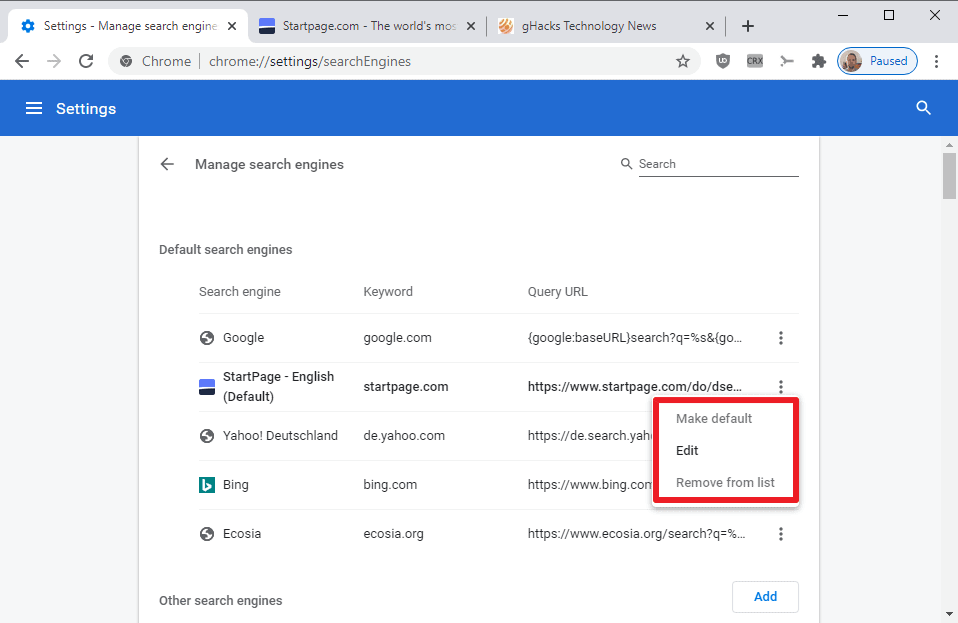This image is a detailed screenshot of a user's settings page within their Google Chrome browser. The user has three browser tabs open: the settings page, Startpage.com, and GHacks Technology News. The Chrome search bar at the top explicitly indicates the user is exploring "Chrome settings search engines."

Prominently displayed on the screen is the settings navigation bar, a long blue rectangle with the word "Settings" on the left and a magnifying glass icon (representing search) on the right. Below this, the section is clearly labeled with "Manage search engines," "Default search engines," followed by a comprehensive list of available search engines including Google, Startpage, Yahoo, Bing, and Ecosia.

For each search engine, specific details are provided: a keyword (essentially the website's name) and the corresponding query URL. A red box overlay appears around some of these query URLs, containing actionable options such as "Make default," "Edit," and "Remove from list," with "Edit" highlighted in solid black.

At the bottom of the settings list, there's a section labeled "Other search engines," which features an additional button for "Add," allowing the user to input and configure further search engines.